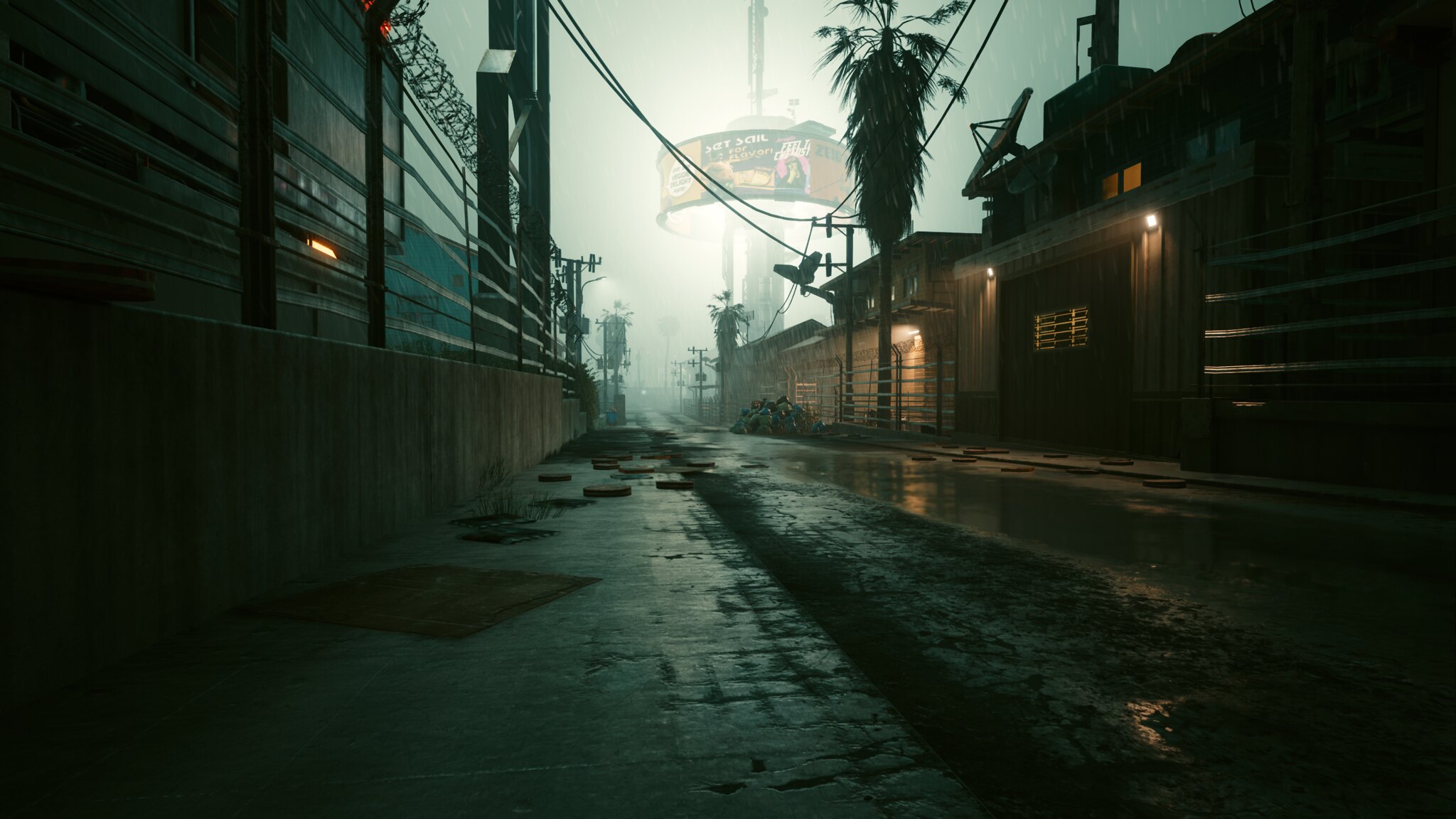The image presents a dimly lit urban scene, seemingly captured in a narrow street or alley. On the left, a dark wall can be observed, adorned with a vertical post and stretching horizontal wires reminiscent of a fence, topped with barbed wire for added security. This wall conceals a substantial, shadowy building looming in the background, further contributing to the mysterious aura of the scene.

The street itself appears wet, as though it has recently rained, with reflections shimmering on the cobblestone sidewalk, which is notably broken and uneven, adding a sense of neglect. On the right, additional fencing stands in front of a series of dark-colored buildings. Some of these buildings feature lit doorways and windows, providing sporadic pockets of light in an otherwise gloomy environment.

In the distance, a couple of palm trees can be faintly discerned, adding a hint of unexpected greenery to the predominantly industrial setting. A large, circular billboard is also visible towards the back, rising above the scene. The sky overhead is a dull, smoggy gray, filled with heavy clouds, enhancing the overall desolate, abandoned feel of the area.